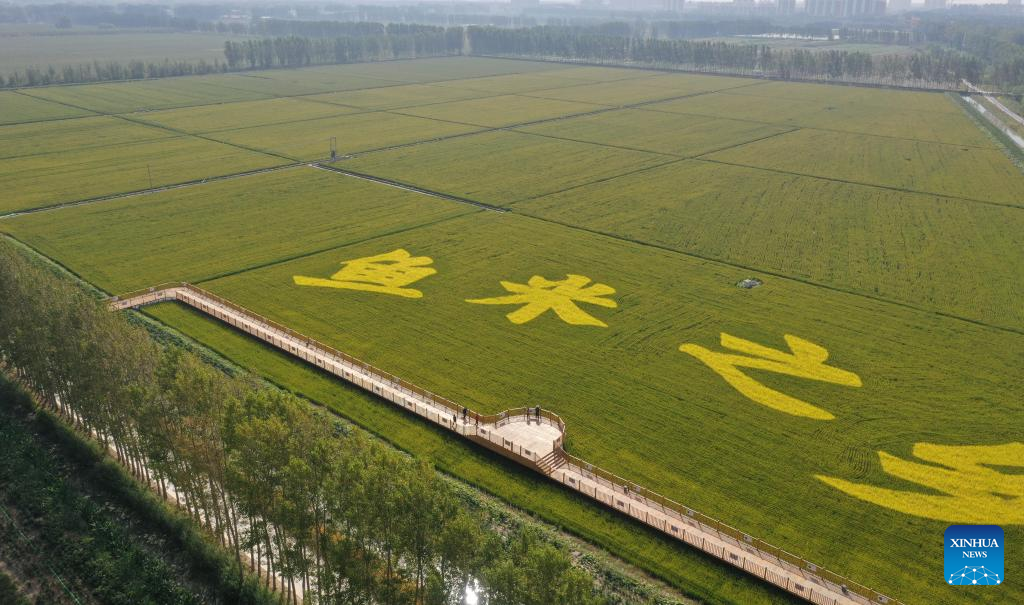The image presents an aerial view of a vast, verdant field divided into a grid of smaller square sections, arranged four across and four up, creating a neat criss-cross pattern. The field is subtly angled, rising from left to right. Prominently at the bottom, four large Chinese characters, rendered in yellow, are clearly visible, contrasting with the green of the grass, which has likely been cut or altered to form these figures. In the lower right corner, a blue box with the text "XINHUA News" in white lettering stands out. At the bottom left, a patch of grass and a tree line extend from the center to the left, intersecting with a cement walkway. This walkway, populated by people who appear tiny against the vastness of the field, zigzags diagonally from the bottom right to the middle left, featuring a rounded, white-lookout deck with a brown railing at its midpoint. In the far distance, another line of tall, slender trees marks the edge of the expansive field, suggesting a serene nature area designed for public enjoyment.